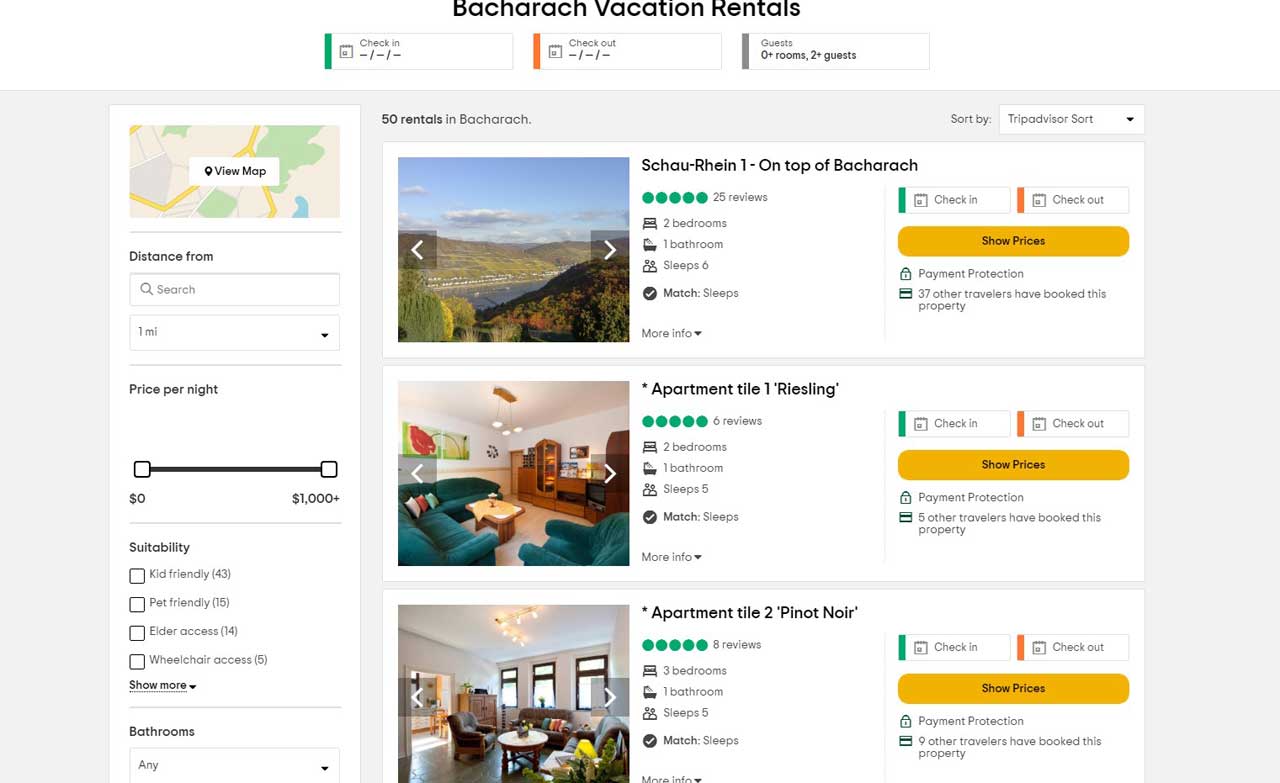**Caption:**

This image showcases a screenshot of Batch RH Vacation Rentals' online platform. At the top, set against a white background, the company's name is prominently displayed in black letters. Beneath, colored bars in shades of green, orange, and gray, each paired with a white bar, add a pop of color.

The main background of the screen has a light gray hue. On the left side, within a white menu, various features and filters can be seen. At the top left corner, there's a clickable "View Map" option. Directly below is the "Distance From" filter with a search bar currently set to "1 mile." A price per night slider allows adjustments from $0 to $1,000. Additional filters include "Sustainability," which highlights options for kid-friendly, pet-friendly, elder access, and wheelchair access accommodations, with a "Show More" option available.

Further down, there's a filter for "Bathrooms" with an adjustable menu set to "Any." On the right side, a gallery presents images of different vacation rental options. The first image features a scenic view of hills blanketed in trees with a body of water in the valley. The second image captures the interior of a room furnished with a teal-colored couch and chair, complemented by a brown coffee table. The third image showcases another room's interior setup with various pieces of furniture.

To the right of these images, the listings' details and reviews can be seen, along with options for users to "Show Prices" and input their "Check In" and "Check Out" dates.